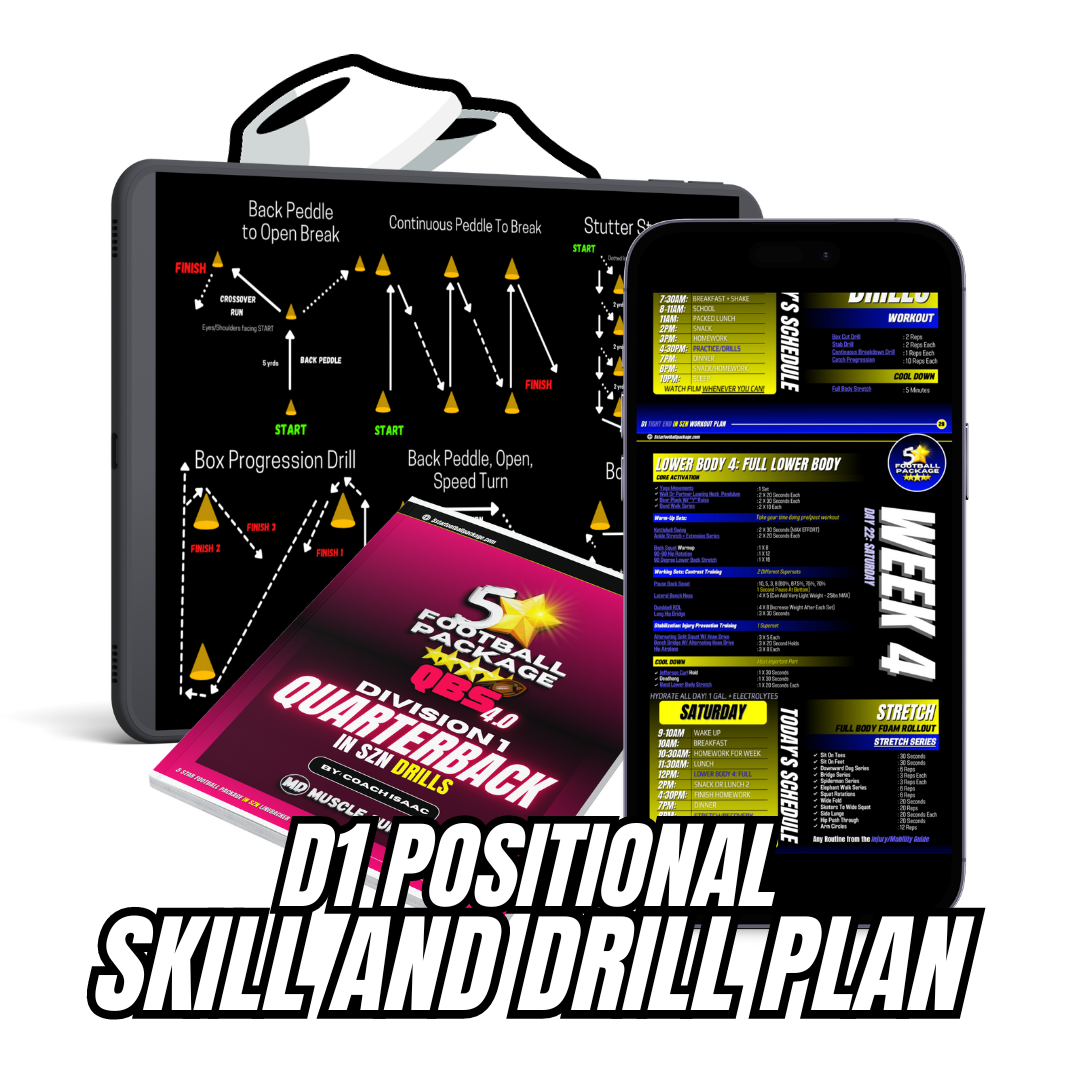The product photograph features a generic 3D-rendered tablet and smartphone displaying an application titled "D1 Positional Skill and Drill Plan," which offers workouts and sports drills for football. Both devices highlight different aspects of the app, with the phone screen displaying a segment labeled "Week 4" and showcasing blue, yellow, and black colors, while the tablet illustrates various training routes. Positioned between the devices is a 3D-rendered book labeled "Five Star Football Package," featuring a yellow star above the text and partially obscuring a fifth star at the bottom. All elements are set against a solid white surface and background, emphasizing the products independently, suitable for commercial use in online stores, catalogs, or websites.